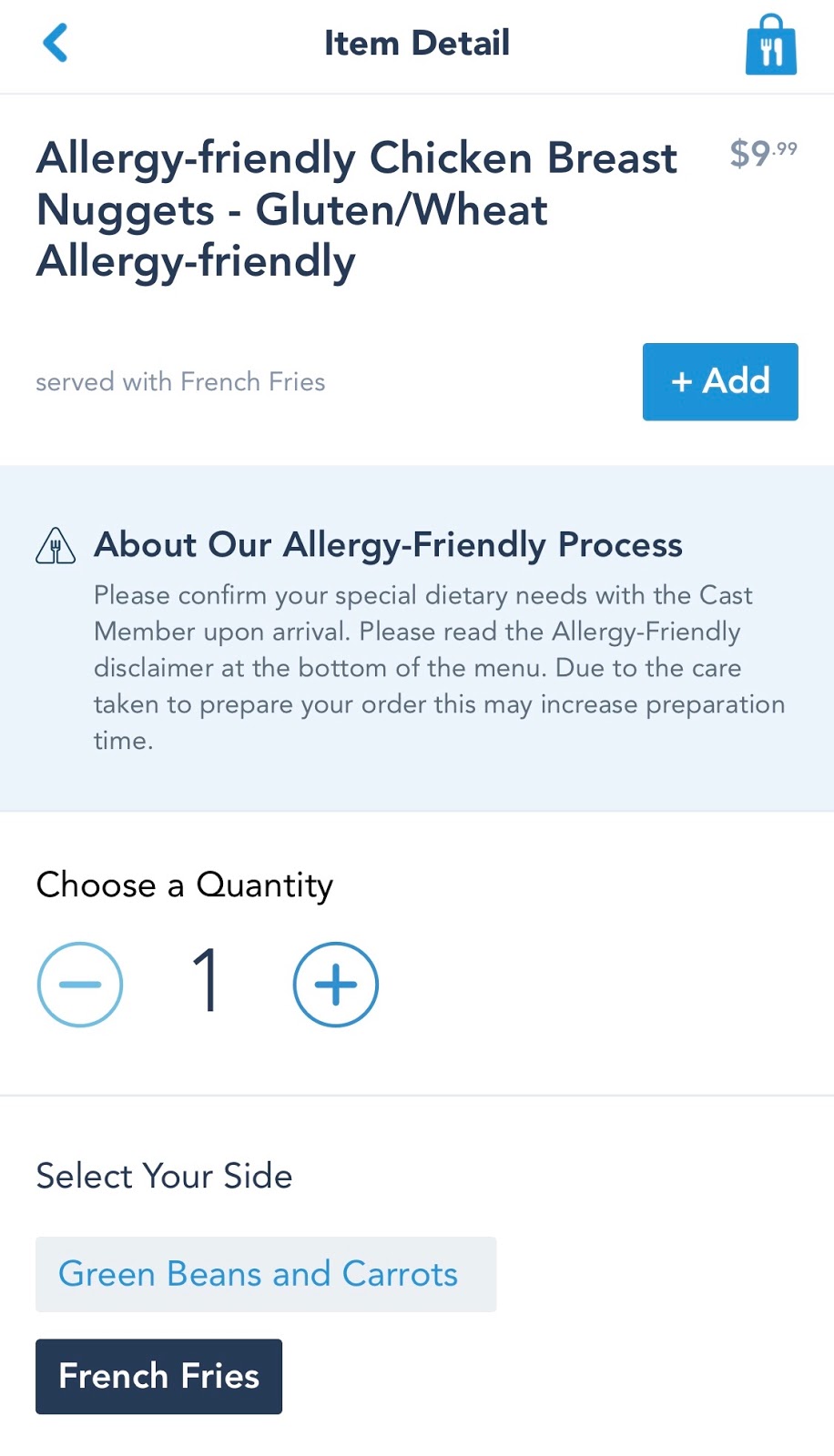This screenshot captures the process of ordering food from an online menu. At the top, the header reads "Item Detail," with a left-facing arrow on the left side for navigation. On the right, there's an image of a blue bag filled with white utensils, which serves as a cart button. Below the header is a gray dividing line.

The main content begins with the text "Allergy-Friendly Chicken Breast Nuggets - Gluten/Wheat Allergy-Friendly $9.99" in black lettering. Directly below, a description notes that the meal is "served with French fries." To the right of this text is a prominent blue rectangle with white lettering that says "Add," which allows users to add the meal to their cart.

Further down, there's a light blue rectangle containing information about the establishment's allergy-friendly process. It advises customers to confirm their special dietary needs with a cast member upon arrival and to read the allergy-friendly disclaimer at the bottom of the menu. It also mentions that the specialized preparation may increase preparation time.

Below this informational section is an area where users can choose the quantity of their order, with a subtraction symbol on the left and an addition symbol on the right. The default quantity is set to one. Finally, there's an option to select a side dish, offering a choice between "Green Beans and Carrots" or "French Fries," with "French Fries" currently highlighted as the selected option.